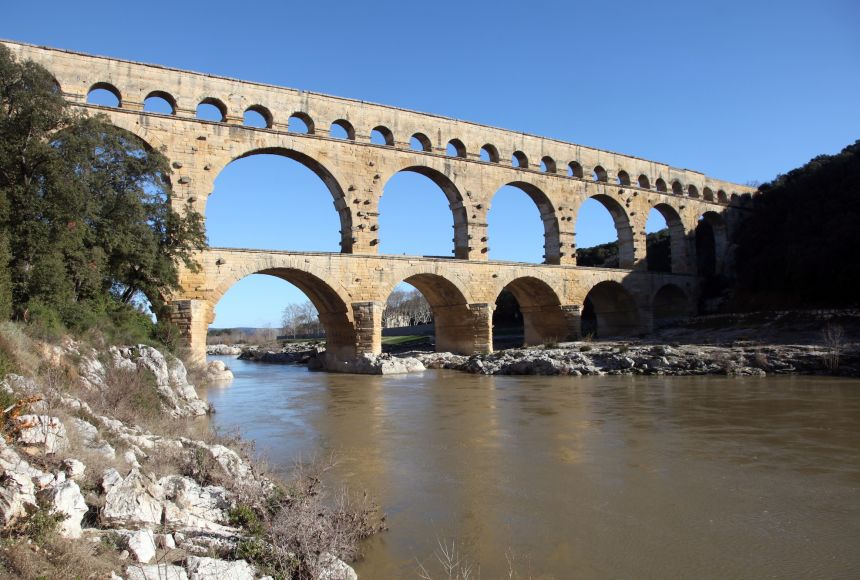The image depicts a remarkably well-preserved Roman-style aqueduct, possibly akin to the Pont du Gard, crossing a broad, rocky river. The aqueduct, constructed from tan and yellowed stones, features a three-tier structure of arches. The bottom and middle tiers have wide, large archways, while the topmost tier consists of much smaller arches. The river below appears murky, with dark brown water that reflects the clear, blue sky above. On the left bank, the rocky shore is dotted with scraggly brush and brambly shrubs, giving an autumn feel, while both banks show small trees and foliage. The aqueduct extends from a hill on the right, seamlessly integrating into the rugged landscape, with empty spaces suggesting the ability to carry water, and possibly even pedestrian traffic. The scene is set against a backdrop of a vivid, cloudless sky, highlighting the timeless architectural legacy of this historical structure.